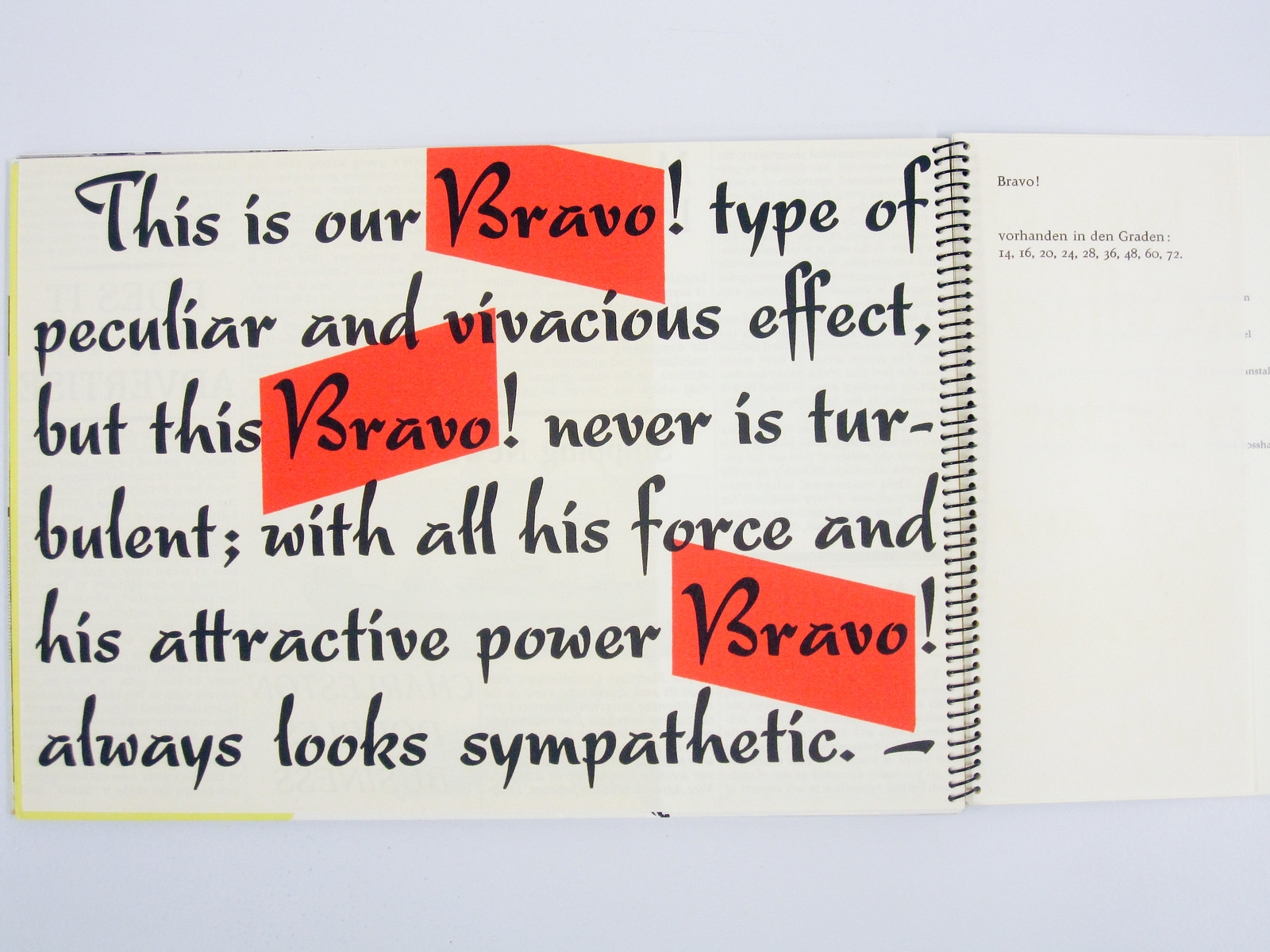This wide rectangular image depicts an open book, laid on a completely white surface, featuring a metal black wire binding positioned closer to the right side. The book appears to be a font specimen booklet with an off-white colored page on the left, bordered in yellow. The detailed text on the left page is presented in a large, bold, and black font that reads: "This is our Bravo type of peculiar and vivacious effect, but this Bravo never is turbulent. With all his force and his attractive power, Bravo always looks sympathetic." The word 'Bravo' appears multiple times, each instance marked by an exclamation point and highlighted by a red skewed rectangle behind it. The right page of the book is partially cut off, but it shows smaller print, including the word 'Bravo' and some German text along with numbers listed beneath it. The overall presentation of the book seems to blend elements of handwritten and gothic styles, showcased through its spiral binding and distinctive typography.